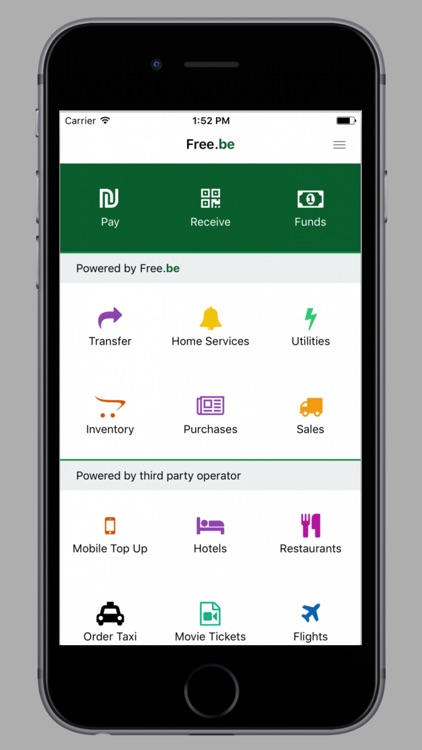The image is a detailed screenshot featuring a black iPhone centered against a gray background. Surrounding the iPhone is a gray frame visible on all sides - top, bottom, left, and right. The phone's screen is on, showcasing various interface elements. 

At the very top of the screen, a white status bar is present. On the left side of this bar, the word "Carrier" is displayed alongside a Wi-Fi icon, indicating an active internet connection. Centrally positioned within this bar is the time, shown as 1:52 PM. On the far right, a battery icon indicates the phone's current power level.

Moving downwards, below the white status bar, the word "Free.B" appears prominently in bold text. Directly beneath this is a green banner extending across the screen. The left side of the banner features the word "Pay" in white text, while the right side reads "Receive" next to "Funds," which is accompanied by an icon of a dollar bill above "Funds."

The lower portion of the screen has a white background section. Within this section, from left to right in blue text, the words "Transfer," "Home," "Services," and "Utilities" are displayed, indicating various available options or sections within the application.